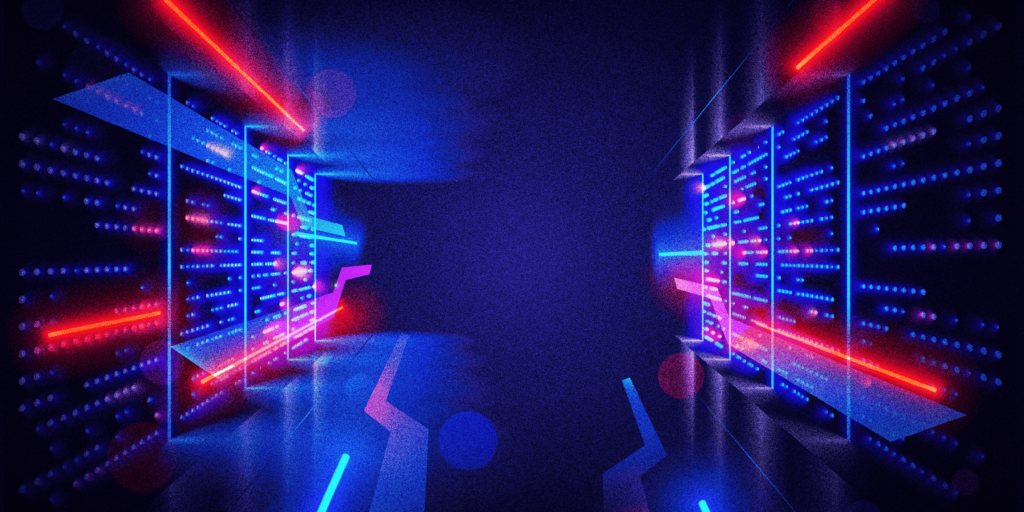The image is a dark, futuristic server room predominantly colored in shades of blue, featuring numerous computer servers arranged along the left and right walls. These servers are adorned with blinking neon lights in red and blue, creating a laser-like effect that gives the room a high-tech, almost cybernetic ambiance. The floor is particularly striking with its shiny, geometric design incorporating blue and red shapes, mirroring the colors and patterns of the walls and ceiling such that they blend seamlessly together. This cohesive color scheme and the room's overall layout evoke a sense akin to a stylized digital stock art often used for technology-related themes. The scene is reminiscent of a corridor lined with imposing technology, similar to a sci-fi movie set, leading towards a focal point – a rectangular shape in the center of the image – creating an almost cinematic pathway through the heart of this advanced computer system.